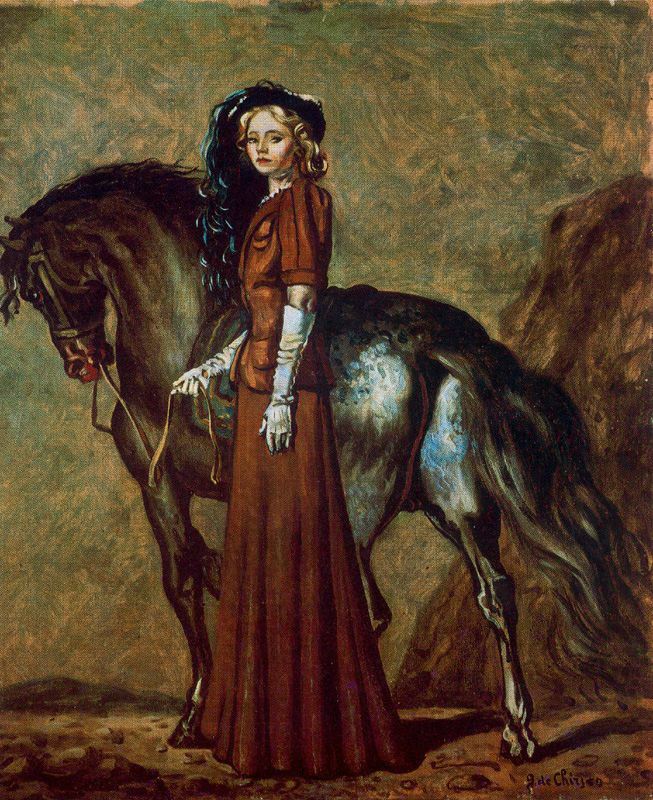This hand-painted image features a sophisticated woman, standing slightly to the left of center, next to a brown horse with hints of white and blue on its coat. She has shoulder-length wavy blonde or brown hair and is dressed in a long brown dress, complemented by long white gloves and a black hat. Her red lipstick adds a touch of elegance to her poised demeanor as she holds the tan reins of the horse in her right hand. The backdrop is a greenish-brown hue, suggesting an outdoor setting, while the ground beneath them is dirt with scattered brown stones. Near the woman, on her right, lies a rock. The painting is signed by the artist in the bottom right corner.